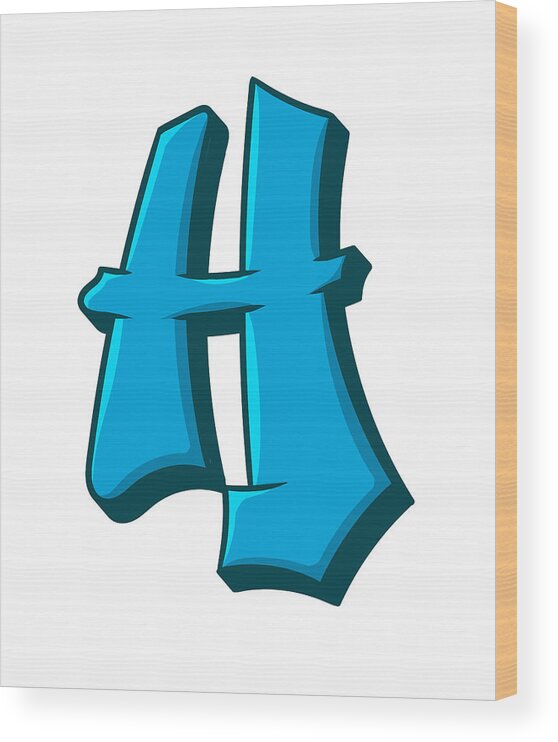The image features a framed art piece resembling a wall hanging, with a wooden frame surrounding a white canvas. Dominating the composition is a large, graffiti-style letter "H" rendered in shades of light and medium blue. The letter is outlined and shadowed to give it a 3D effect, making it appear as if it is popping out from the canvas. The background behind the H is a darker blue, adding depth to the artwork. The canvas itself has a noticeable lined texture running through the H, and a yellowish edge is visible on the right side, further emphasizing the frame's construction. Overall, the piece is a striking example of graffiti art presented in a gallery-like format.